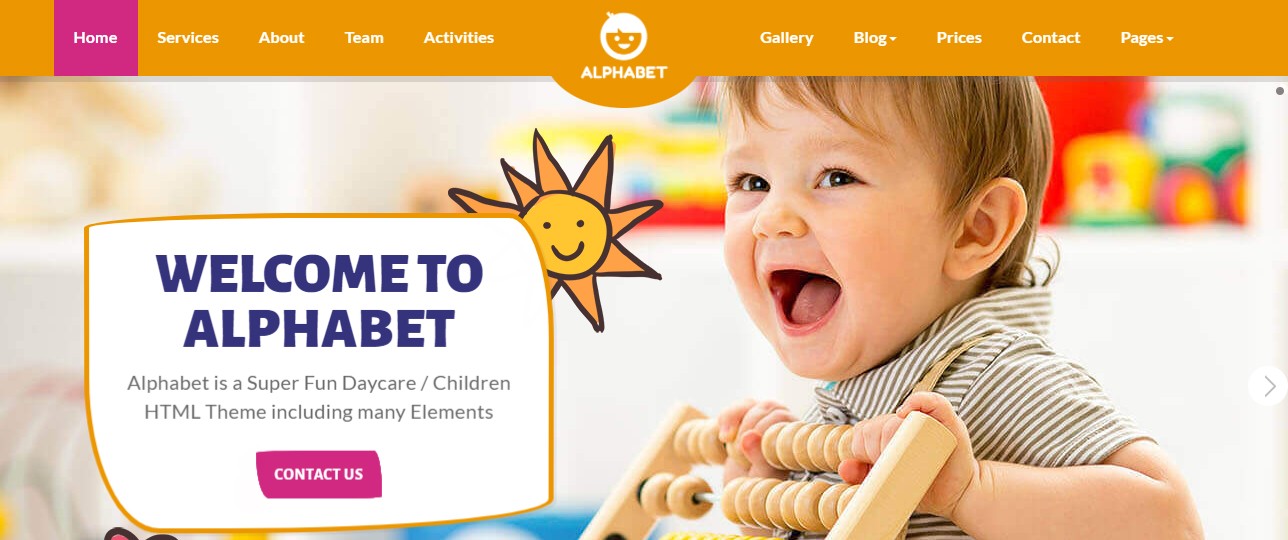The image features a vibrant interface design with a distinct orange rectangle at the top. Towards the left side, there is a prominent pink square labeled "Home." Across the orange banner, one can find additional labels including "Services," "About," "Team," and "Activities." Attached to the bottom of this rectangle is a partial circle, which features a face design, accompanied by labels such as "Alphabet," "Gallery," "Blog" (with a downward-pointing arrow), "Prices," and "Contact Pages" (also with a downward-pointing arrow).

Central to the image is a cheerful visual element: a drawing of a sun with a smiling face, alongside a child holding a toy and dressed in a striped, gray and white shirt. The child shares the focal point with a somewhat irregularly shaped, hand-drawn rectangle in blue, containing the welcoming message: "Welcome to Alphabet." Below this, it reads: "Alphabet is a super fun daycare/children HTML theme including many elements."

Additionally, there is a slightly crooked pink rectangle with the words "Contact Us" in white. Behind the child's head, a few toys are visible but they remain indistinct due to blurriness.